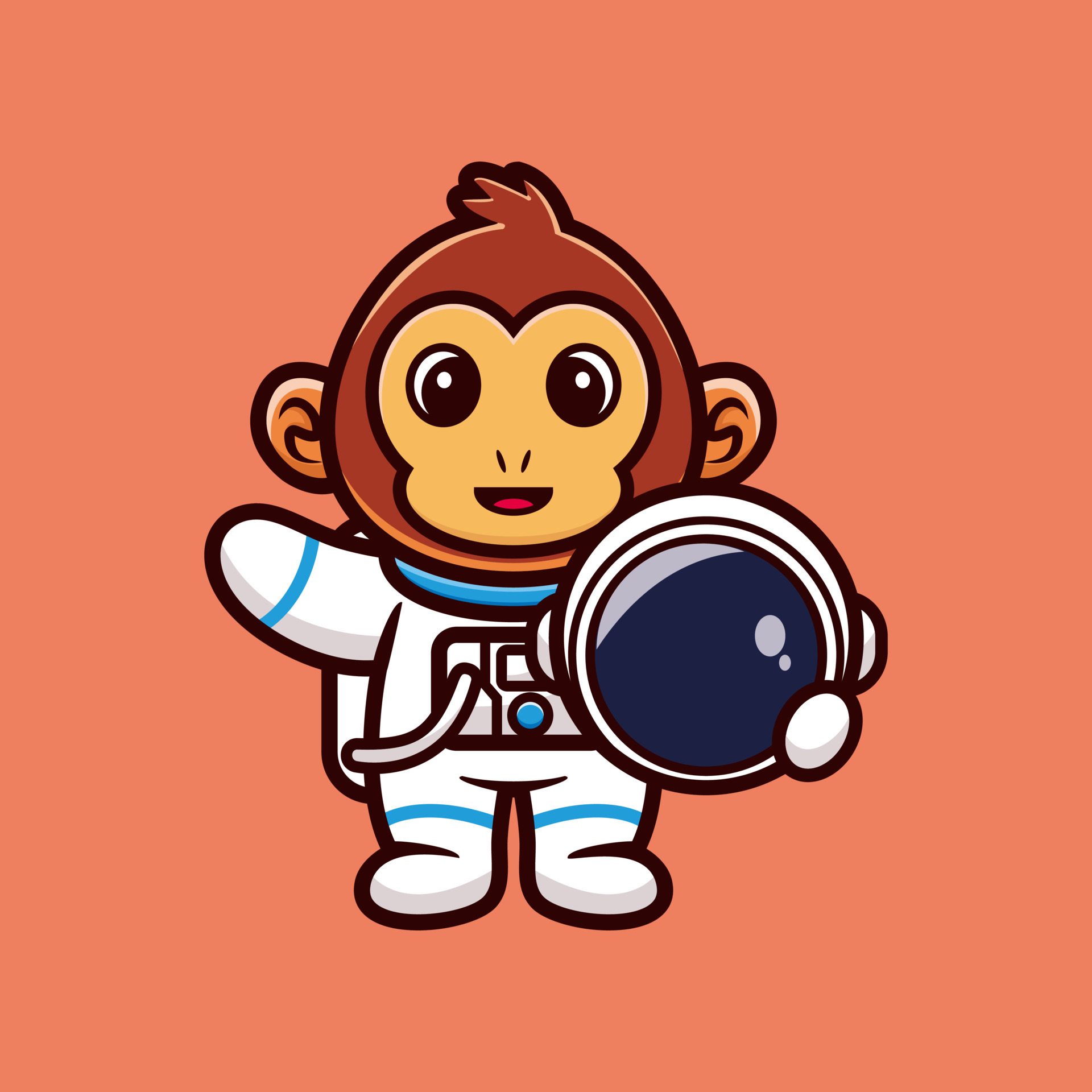This whimsical illustration depicts a small, cartoonish brown monkey with tan ears and face, standing against a solid peachy orange background. The monkey, characterized by its giant black eyes with white dots and a slight smile, appears to be happily waving with its right arm while holding a space helmet with a blue visor in its left arm. The monkey's astronaut suit is predominantly white with blue details, including a blue collar, blue stripes on the arms and legs, and blue trim around the neckline, wrists, and ankles. There's a noticeable square on the suit's chest, possibly indicative of a connection point for air or life support, and a backpack attached to the back completes the monkey's space explorer look. The background is plain and unpatterned, emphasizing the simplicity of this charming and cute illustration, reminiscent of a character from a children's book.